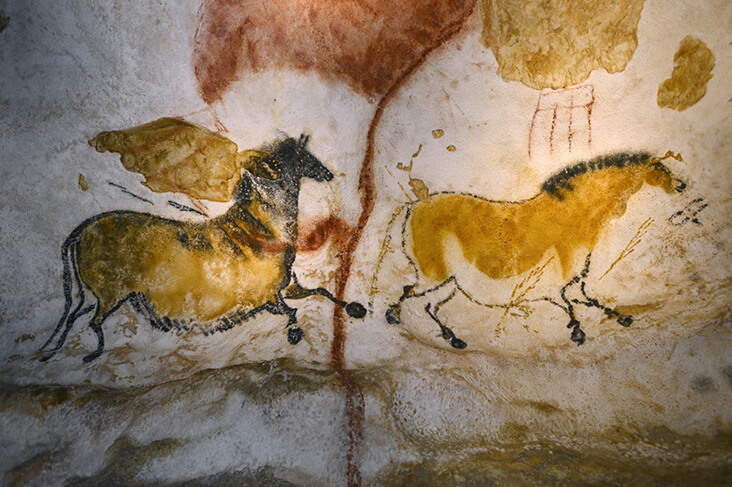This image captures an ancient cave painting, likely inspired by the famous Lascaux, France site. The artwork is set against a rocky wall with a distinct yellowish-brown hue accentuated by some white and dark veining textures. Notably, a maroon red seam runs down the middle, with a red splash extending to the side, which may either be part of the rock's natural formation or integrated into the painting. The central figures are two black-outlined, ochre-colored horses, each with notably wide bellies and thin, black legs, positioned sideways as if in motion. The horse on the left, adorned with more detailed black features, appears to be galloping, while the one on the right seems to be walking or running in a different gait. Above the horses and interspersed around them are various cave painting symbols and patterns, adding to the enigmatic nature of the scene. The overall image, possibly taken with flash photography despite typical restrictions, highlights the intricate and historic artistry etched directly onto the cave's surface.